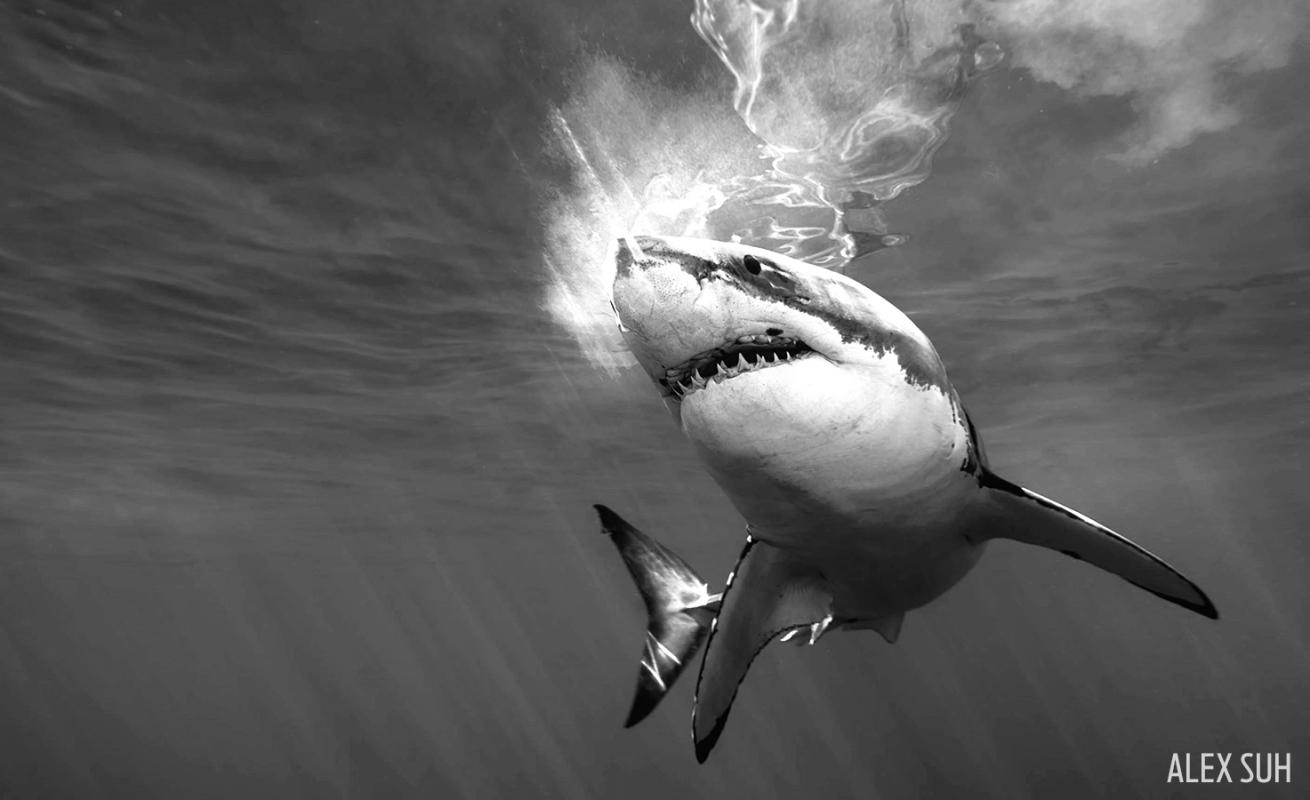This black-and-white underwater photograph, presumably taken by Alex Suh (as credited in white letters at the bottom of the image), captures an awe-inspiring great white shark in its natural habitat. The shark, depicted with striking detail, glides with its large back fin and two forward fins clearly visible. Its body features a pronounced contrast: a completely white underside from the pointed nose down to the chest, with the rest of its body in various shades of gray and black, including white stripes on its fins and some white dots on the dorsal fins. The creature's mouth is slightly open, revealing rows of very sharp, large teeth, with two particularly notable at the bottom. The skin around its eye has dark markings running from the nose to the fins, and the tail exhibits a pattern of black striping. The image is taken from a slightly lower angle, allowing viewers to also glimpse rays of sunlight filtering through the water, creating a lighter area above the shark against the otherwise dark ocean depths. In the background, waves and bubbles enhance the dynamic sense of movement, giving life to this mesmerizing underwater scene.